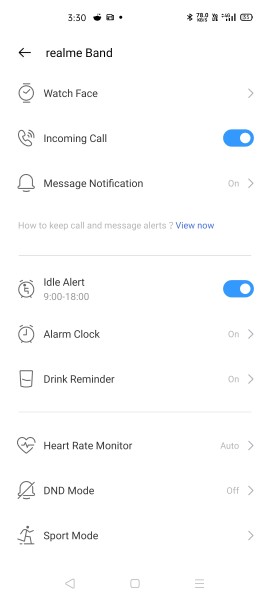The screenshot appears to be taken from a cell phone, displayed on a white background. At the top, in black text, it indicates the time "3:30" accompanied by a series of icons on the right side, showing Bluetooth, LTE, a 4G cell signal, and a 35% battery level.

Below this header, the text states "Realme band" with "Realme" in lowercase and "Band" starting with an uppercase letter B. There is then a left-facing arrow symbol next to this heading.

Further down, the interface shows various options:
- "Watch face" accompanied by a right-facing arrow.
- "Incoming call" settings turned on.
- "Message notification" settings turned on, also accompanied by a right-facing arrow.
- A link titled "How to keep call and message alerts?" with a blue "View Now" hyperlink.

The next section lists:
- "Idle alert" scheduled from 9:00 to 18:00, turned on.
- "Alarm clock" turned on, with a right-facing arrow.
- "Drink reminder" turned on, with a right-facing arrow.
- "Heart rate monitor" set to auto, with a right-facing arrow.
- "DND mode" (Do Not Disturb) turned off, with a right-facing arrow.
- "Sport mode" also linked to a right-facing arrow.

At the bottom, faded text or shading encloses an arrow pointing to the right, a square icon in the middle, and a stack of three horizontal lines, possibly representing a menu icon.